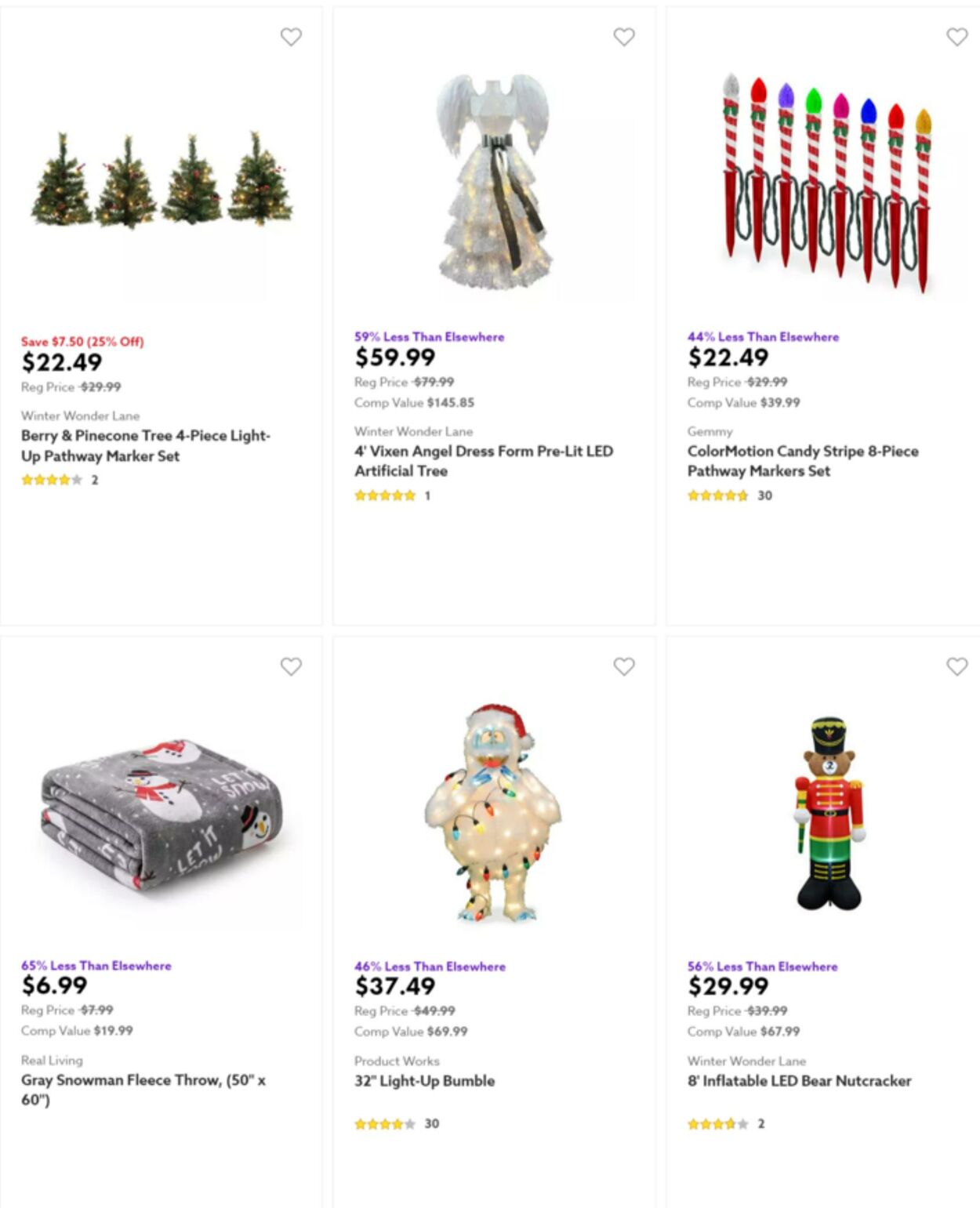This festive image showcases an array of six Christmas-themed items arranged in two rows. Let's dive into each item in detail:

**Top Row:**
1. **Burying Prince Tree Four Piece Light Up Pathway Marker Set:** This set features four small, horizontal Christmas trees crafted to light up your pathway. Each tree is adorned with festive decor and priced at $22.49, discounted from the regular price of $29.99.
2. **4-inch Fixing Angel Dress from Pre-Lit LED Artificial Tree:** This elegant angel tree topper stands modestly at 4 inches tall. It is dressed beautifully and includes pre-lit LED lights to add a magical glow to your Christmas tree.
3. **Color Motion Candy Stripe Eight Piece Pathway Marker Set:** This vibrant set includes eight pathway markers, each designed with colorful stripes that exhibit a lively motion pattern, perfect for guiding guests to your doorstep during the holidays.

**Bottom Row:**
1. **Gary Snowman Feliz Throw:** Measuring 50 by 60 inches, this cozy throw features a cheerful snowman named Gary who is wishing everyone a "Feliz Navidad." Priced at an affordable $6.99, it's perfect for snuggling up during the chilly holiday season.
2. **32-inch Light Up Bumble:** Standing at a substantial 32 inches, this eye-catching decoration features a character named Bumble, who lights up to spread joy. Priced at $37.49, Bumble is sure to be a standout piece in your holiday decor.
3. **8-inch Inflatable LED Bear Nutcracker:** This delightful inflatable bear, dressed as a nutcracker, stands at 8 inches tall. It is illuminated with LED lights and priced at $29.99, making it an enchanting addition to any festive display.

These items collectively offer a diverse range of holiday decor options, from pathway markers to cozy throws, ensuring a festive and welcoming atmosphere.